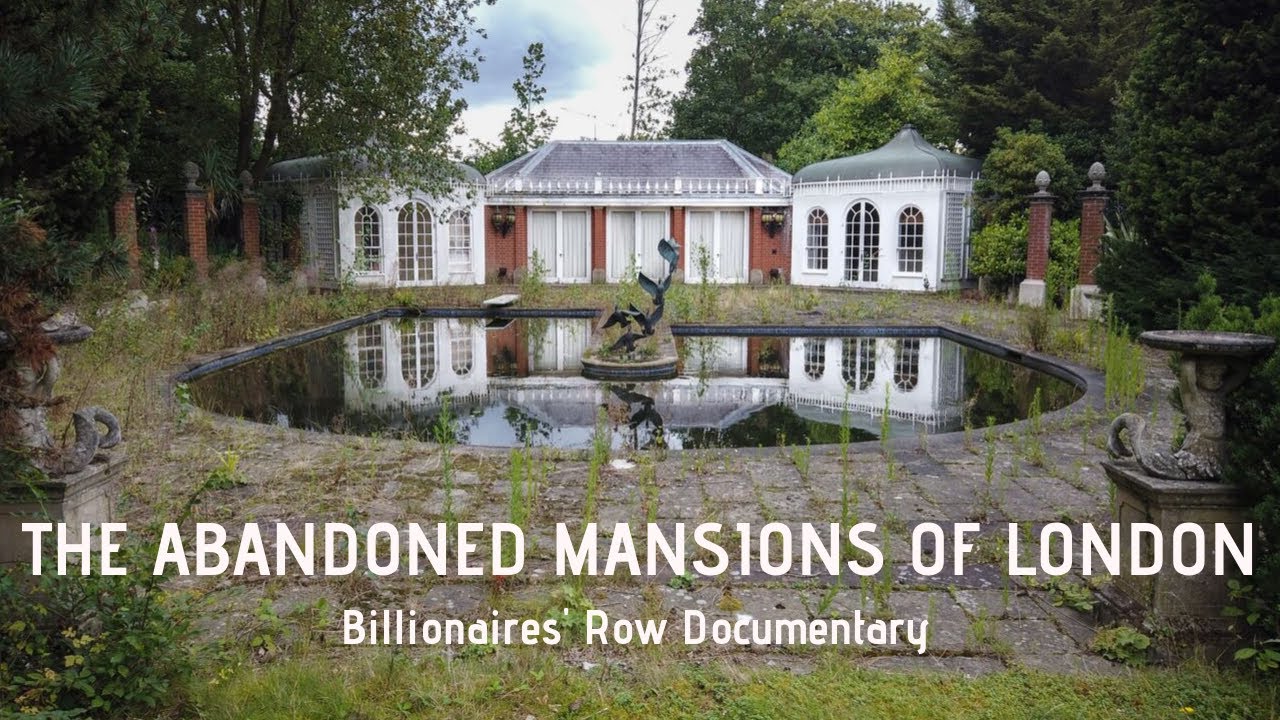This photograph, captioned "The Abandoned Mansions of London, Billionaires Row Documentary," depicts a forlorn pool house or the rear facade of a larger house, with neglected grounds overtaken by grasses and bushes. Central to the image is a large, unkempt pool with a distinctive U-shaped bird statue in the middle, implying it may have once functioned as an ornate fountain. Surrounding the pool are overgrown stone walkways and tiles with two ornate columns holding mermaid sculptures on either side, further indicating the site's former opulence. The house itself features a red brick central section with three French door windows, each framed by white panels. On either side of the central structure are white buildings with arched windows and matching French doors. The decaying grandeur of the scene is accentuated by tall trees and dense foliage reclaiming the space, emphasizing the desolate and deserted nature of this once-glorious estate.